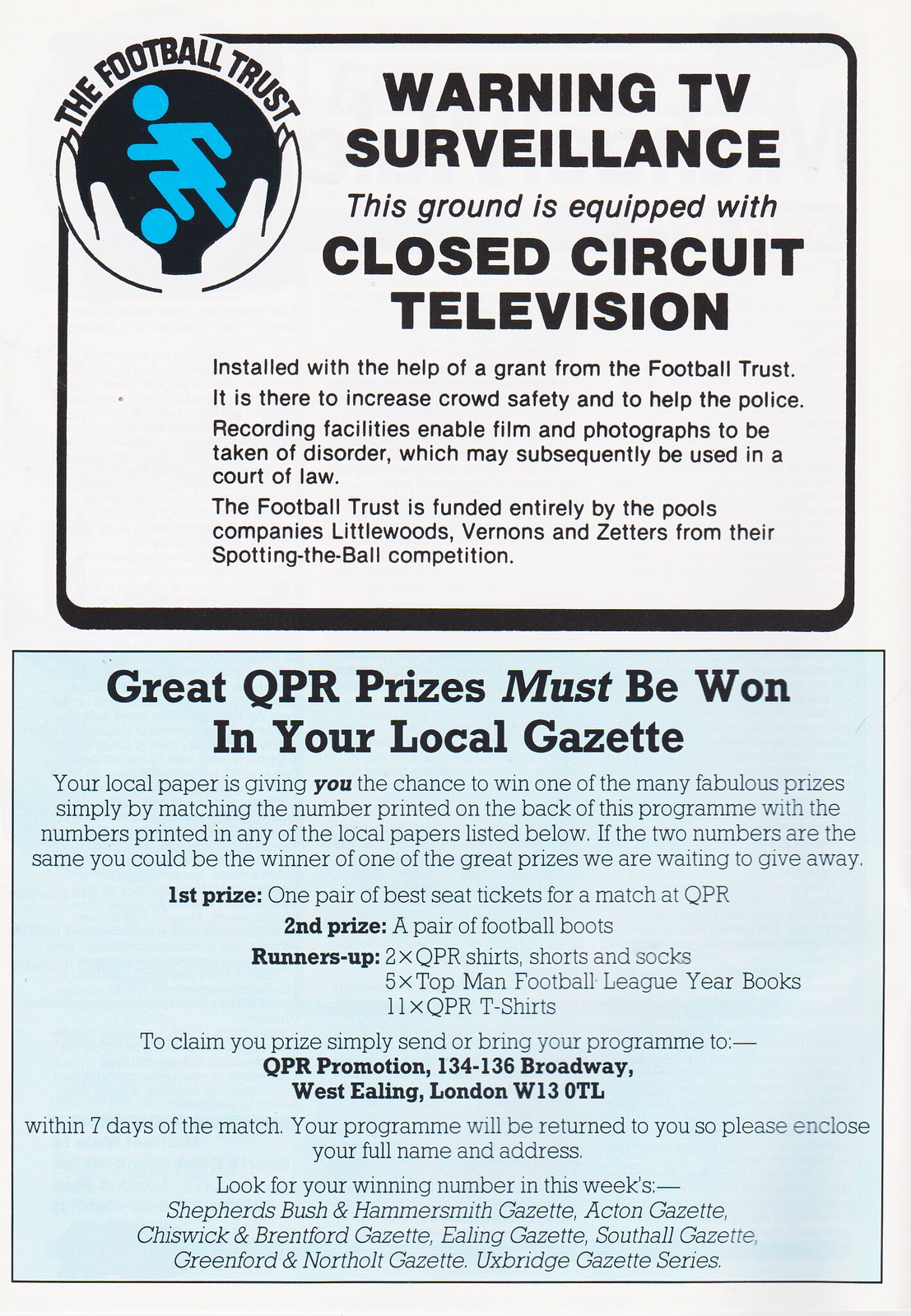This image features a bifold pamphlet with two distinct parts, promoting the Football Trust and a prize competition. The top section is headlined "The Football Trust" and illustrates two hands lifting a large ball containing a blue design of a soccer player set against a black background. It prominently displays a "Warning TV Surveillance" notice, informing the reader that the ground is equipped with closed-circuit television (CCTV) to enhance crowd safety and assist the police, thanks to a grant from the Football Trust. The text emphasizes that these facilities allow for film and photographs to be used in court to combat disorder. The Football Trust is funded by the Pools Company's Littlewoods, Vernons, and Zetters, through their Spotting the Ball competition.

The bottom section advertises, "Great QPR Prizes Must Be Won in Your Local Gazette," and explains a contest organized in collaboration with local newspapers. Participants can win fabulous prizes, such as best seat tickets for a QPR match, by matching numbers printed on the back of their program with those listed in the participating local papers. The pamphlet thus serves dual purposes: to caution attendees about surveillance for safety and to entice them with an opportunity to win exciting prizes through their local Gazette.